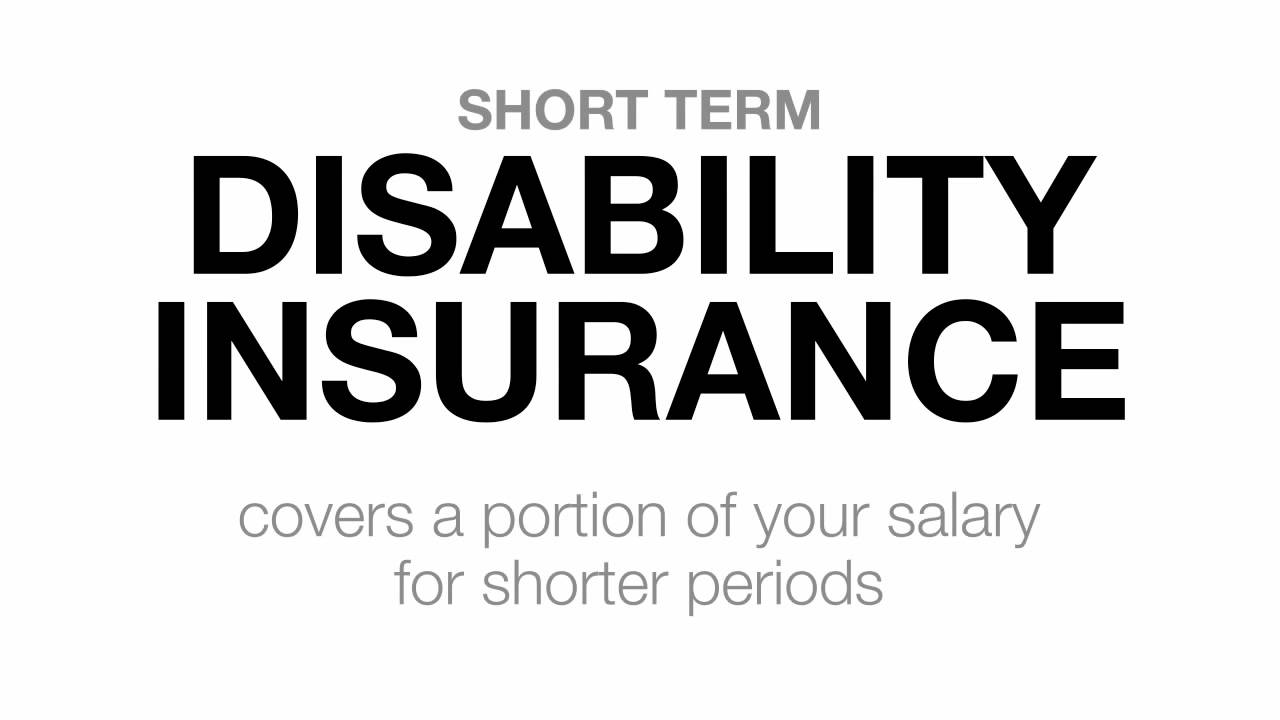This horizontal rectangular image features a centered composition of text on a pure white background. At the top, in smaller light gray uppercase letters, is the phrase "SHORT-TERM." Below this, two large bold black lines dominate the center of the image, reading "DISABILITY" and "INSURANCE" respectively, both in all capital letters. Beneath "INSURANCE," there's a noticeable white space, followed by two lines of smaller, thinner gray text that state, "covers a portion of your salary" and "for shorter periods." This image serves as a straightforward advertisement for a short-term disability insurance program, emphasizing key points with varying font sizes and colors to quickly catch attention and succinctly explain the product.